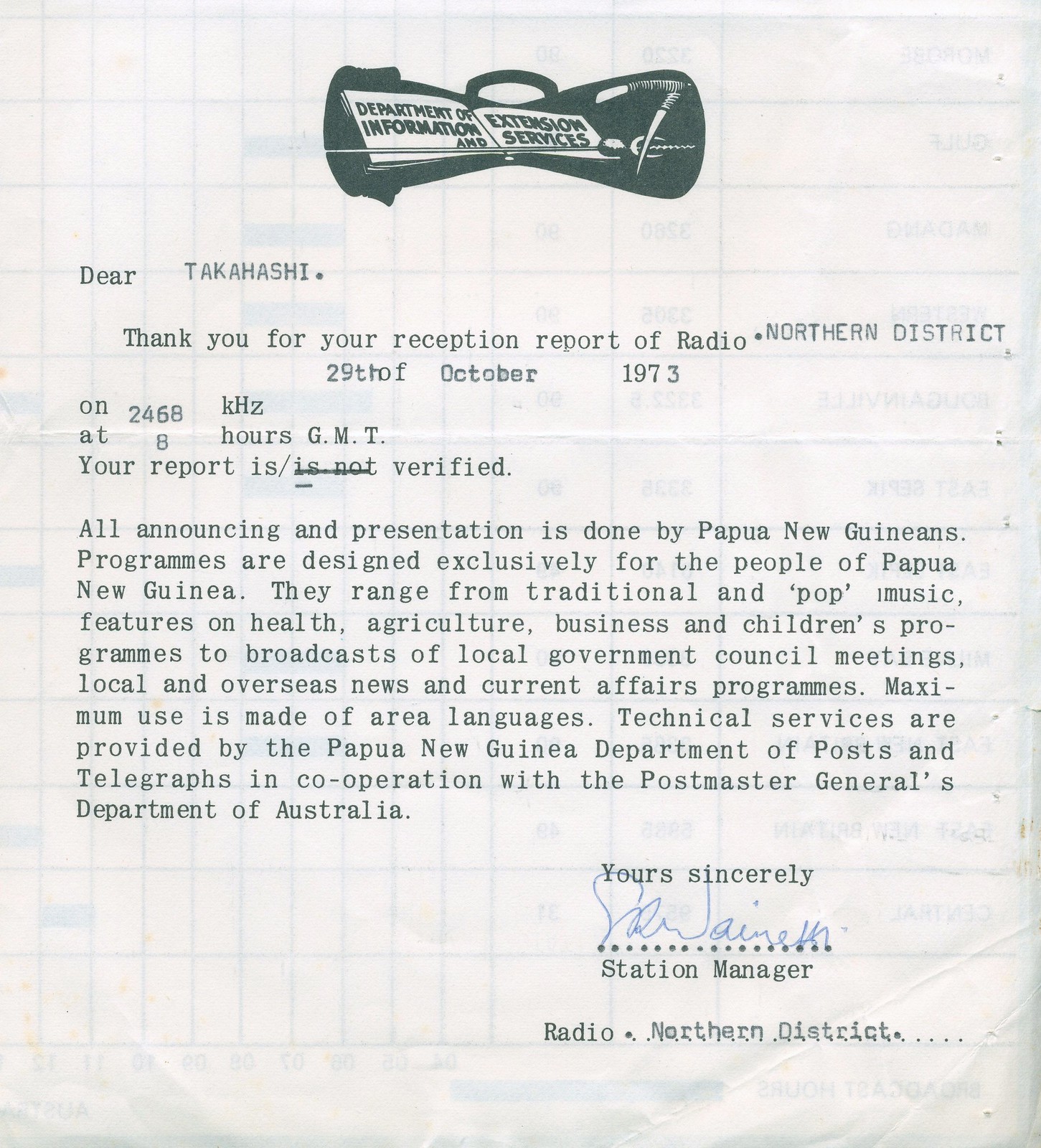The image is a scan of a thin piece of white paper with the text faintly visible from the other side. At the top, centered, there is a black logo resembling a duffel bag and next to it, "Department of Information and Extension Services" is written in black ink. The document, typewritten and dated 29th of October 1973, addresses "Takahashi" and thanks them for their reception report of Radio Northern District on the frequency of 2468 kilohertz at 8 hours GMT, confirming the report as verified. Detailed information follows about the radio station's operations, stating that all announcing and presentation is done by Papua New Guineans. The programs, spelled in British English as "programmes," are designed specifically for the people of Papua New Guinea and include a variety of content such as traditional and pop music, features on health, agriculture, business, children's programs, as well as local government council meetings, local and overseas news, and current affairs. The document mentions that the technical services are provided by the Papua New Guinea Department of Posts and Telegraphs in cooperation with the Postmaster General's Department of Australia. The letter concludes with a handwritten signature in blue pen, underlined with the typed designation "Yours sincerely, Station Manager, Radio Northern District."